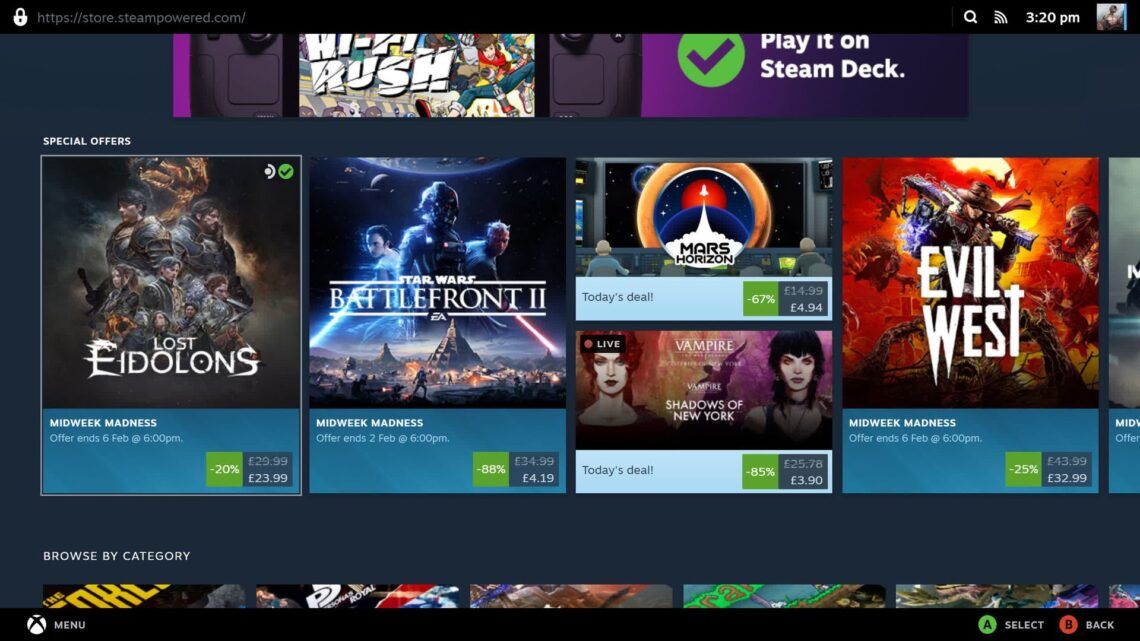In this image, we see what appears to be the main menu of an Xbox interface at first glance. However, closer inspection reveals it is actually a screenshot of the Steam Store webpage, evidenced by the URL "https://store.steampowered.com" displayed at the top left corner next to a white lock symbol, indicating a secure connection.

In the top right corner of the image, there's a profile picture of a user, with the current time beneath it reading 3:20 PM. Additionally, a Wi-Fi icon next to the time shows full signal strength, and a magnifying glass icon indicates a search function.

Dominating the center of the image are multiple game listings, each highlighted with a sale tag. The leftmost game is "Lost Eidolons" with a sale tag indicating a 20% discount. Originally priced at $29.99, the new sale price is displayed as $23.99, with the original price scratched out.

To the immediate right is "Star Wars Battlefront 2," showcasing a significant discount of 88%. The original price is not visible, but the current sale price is prominently marked at $4.19.

At the very top center of the image is an advertisement for the Steam Deck device. Next to a promotional image of the Steam Deck, it reads "Play it on Steam Deck," accompanied by a green checkmark to the left, suggesting compatibility with the device.

This detailed, visual blend of elements distinctly represents a Steam Store page, emphasizing various promotional discounts and highlighting the Steam Deck's compatibility with the featured games.